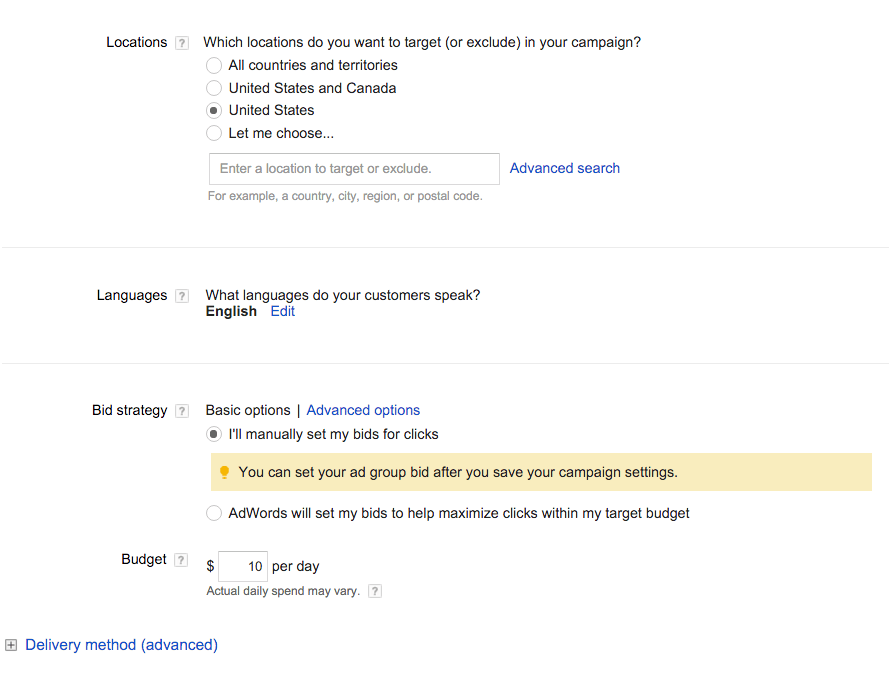This is an image of a location-based web application interface designed for campaign management. The interface allows users to set various parameters for targeting or excluding specific areas. 

- **Location Selection**: The section starts with a question prompting users to define the locations they want to target or exclude in their campaign. Users have options to fill circles beside the following choices:
  - All countries and territories
  - United States and Canada
  - United States only
  - A customizable option to "Enter a location to target or exclude"

  Additionally, there's a "Match Search" feature that assists in refining location choices. In this particular instance, "United States" has been selected, indicated by a filled circle. 

- **Languages**: Below the location options, users can specify the languages they want their customers to speak. The question posed is, "What languages do you want your customers to speak?" with "English" currently selected.

- **Bid Strategy**: This section asks users to choose their bid strategy, with "Basic Options" on the left. The person has selected "I'll manually set my bids for clicks." 

- **Budget**: There is also a section dedicated to setting the campaign budget.

Overall, the interface is structured to guide users through setting essential parameters for their marketing campaign, making it user-friendly and customizable to specific needs.